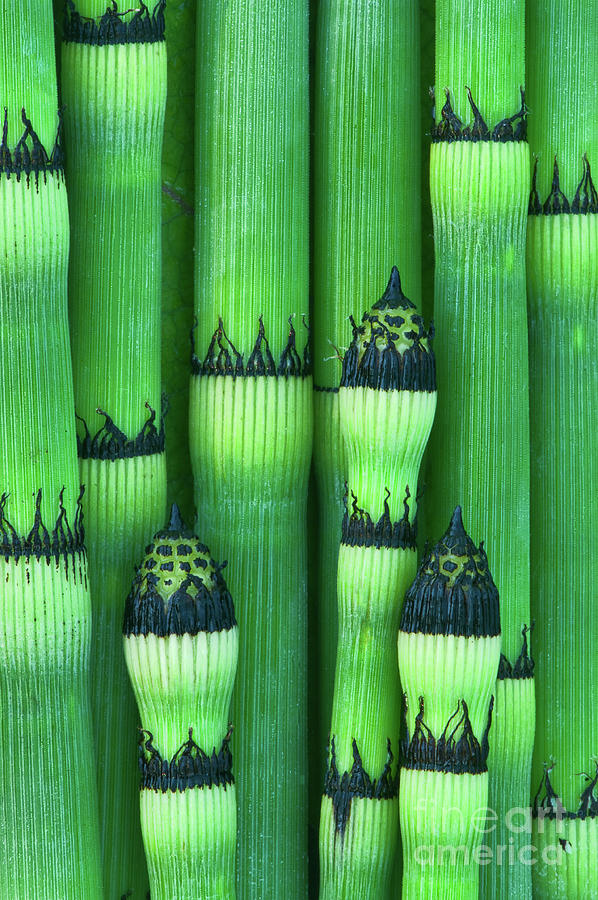The image features a vividly colored, intricate illustration labeled "Fine Art America" at the bottom. Above this label, the artwork portrays a lush, bright green field of tuberous plants, reminiscent of flower beds seen with tulips or other cut flowers. Interspersed among the greenery, a section of stalks bears a resemblance to asparagus. Dotted throughout the scene, dark brown and black peaks emerge from the tops of some shoots, evoking the look of green onions or similarly structured plants. These elements coalesce into a dense, flourishing colony of green tubers, seemingly stacked one upon another in a visually striking arrangement. To accentuate the whimsical nature of the scene, black fringes and architectural forms akin to the domes of the Taj Mahal rise above the verdant field, adding an unexpected and ornate touch to the botanical tableau.